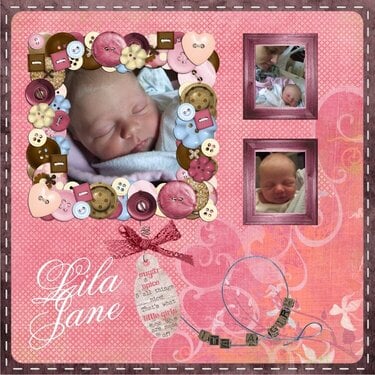The image features an intricately designed birth announcement keepsake, primarily in pink with a brown border accented by white stitching. The central background showcases peach-colored swirls. In the upper left corner, there's a large photo of a swaddled newborn baby, asleep in a blanket, bordered by an overlapping array of buttons in various colors including pinks, yellows, and browns, and in different shapes such as circles, hearts, and crimped button-flowers. To the right, two smaller photos of the baby, also sleeping, are stacked vertically; the top photo includes another child gazing down at the baby, while the bottom solely features the baby's face. Both smaller photos have a framed border simulating pink wood grain. In the lower left corner, elegantly written in cursive, is the child's name, "Lilla Jane." Below this, there’s a tag, possibly containing birth details, although the text is unreadable. In the bottom right, a delicate bracelet announces "It’s a girl."